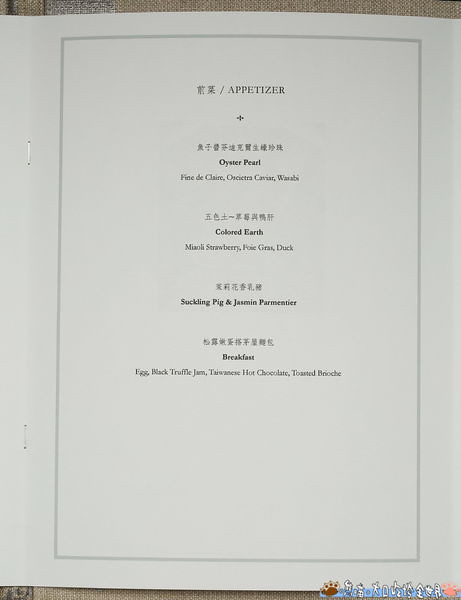A close-up view of the central page of a restaurant menu printed on white paper, secured by two visible staple pins on the left side. The menu features bilingual text, with English and another East Asian language, potentially Chinese or Japanese. At the top of the page, the section is labeled "Appetizer," followed by a list of delectable items. The English names of the dishes include "Oyster Pearl," "Colored Earth," "Suckling Pig," "Jasmine Pomegranate," and "Breakfast." The layout and design offer a glimpse into a curated culinary experience, blending cultural delicacies with descriptive elegance.